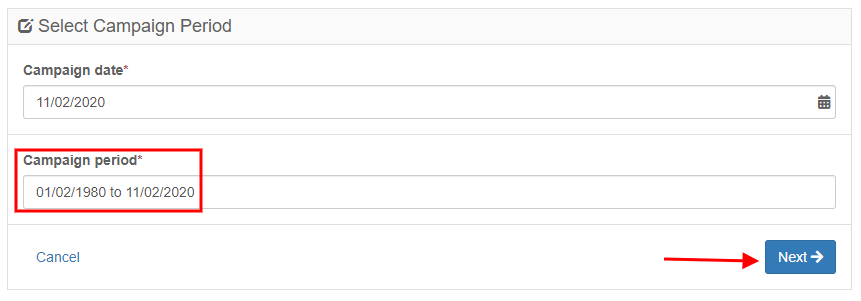This image is a detailed view of a webpage section for inputting campaign information. At the top, there is a light gray banner spanning across the width of the section, with a small square icon on the left labeled "Select Campaign Period." Below this banner, the background changes to white.

The first field is labeled "Campaign Date" in small, bold text, accompanied by an asterisk, indicating it is a required field. Directly below this label is a white input box stretching across the section, containing the date "11/2020." On the right side of this box, there is a calendar icon, suggesting that users can click it to select a different date.

Below this, another required field is labeled "Campaign Period," also marked with an asterisk. In the input box under this label, the range "1980 to 2020" is entered. Both input fields and their labels are outlined in red, indicating a possible annotation or highlight added after the screenshot was taken.

Further down, a thin gray line separates these fields from the navigation options. On the lower left, there is a clickable text labeled "Cancel." To its right, there is a blue "Next" button featuring a right-pointing arrow. A red arrow annotation is placed beside this button, pointing towards it.

This screenshot clearly focuses on the critical areas of form input and navigation within the campaign setup section, making it easy to understand and follow the required steps.